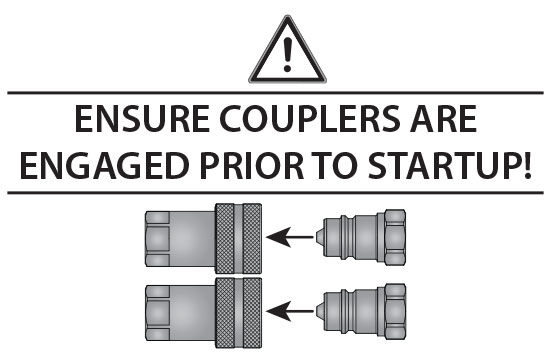The image is an informational graphic set against a stark white background. Dominating the top center is a black triangle with a white center, housing a black exclamation point, serving as a universal caution symbol. Directly beneath this symbol, two rows of bold black text underscore the cautionary message: "Ensure couplers are engaged prior to startup!" The text is framed by horizontal black lines above and below for emphasis. At the bottom of the image, there are two identical coupler systems portrayed in shades of gray and black. On the left, each coupler begins as a short gray cylinder featuring two vertical rectangles dotted with small gray circles. The right-hand couplers taper from a wide base to a narrower end, achieving varied thickness along their lengths. A black arrow directs attention from the tapered end of the right-hand coupler towards the left, suggesting that it should be inserted into the gray cylinder to form a secure connection. These couplers resemble those used in airline or trailer connections, complete with gaskets to prevent leakage.